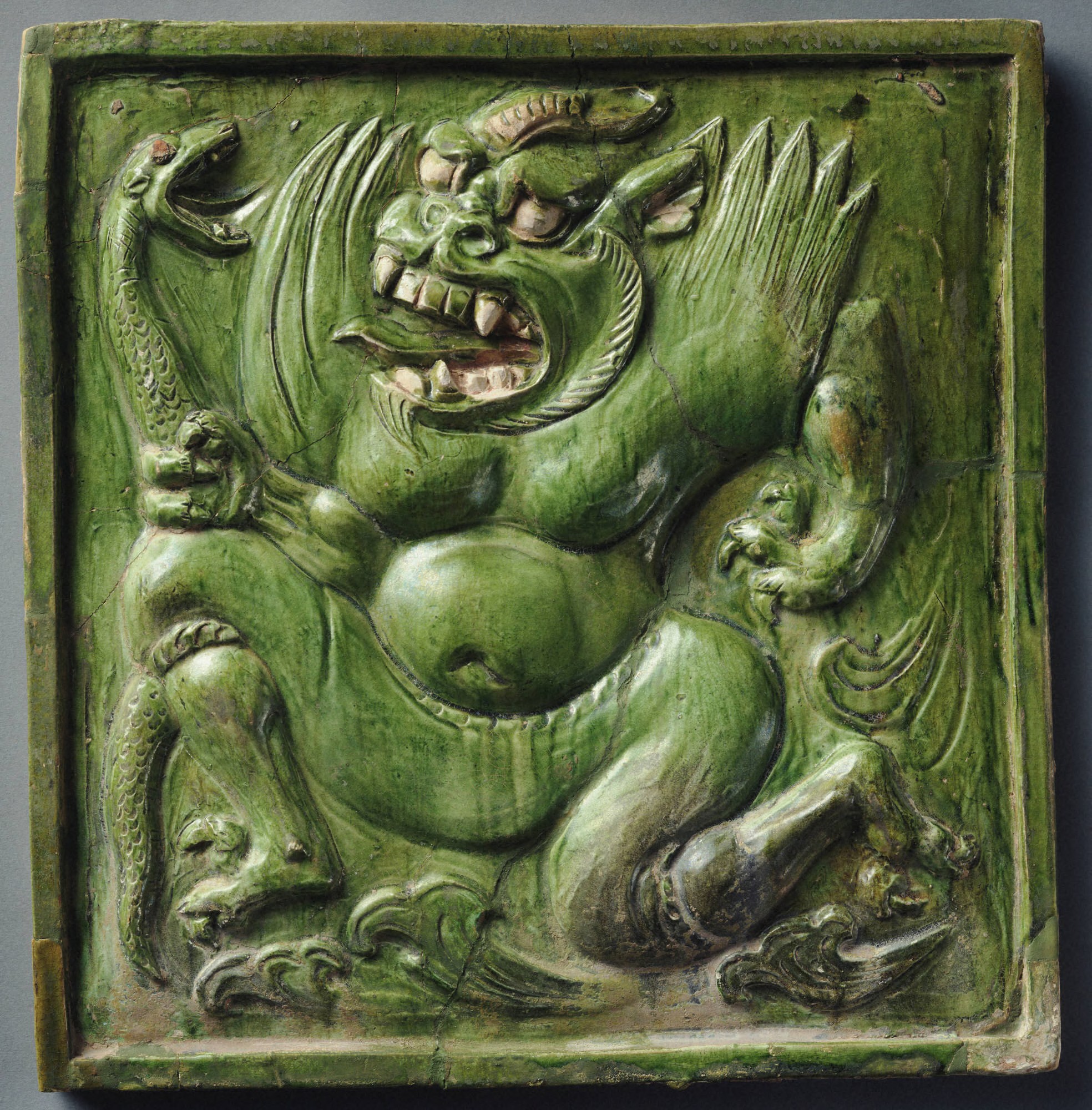The image depicts a square, green-hued carving, framed and mounted on a grey wall, resembling the dimensions of a painting. This elaborate carving, likely made from dyed wood, portrays a heated battle scene between a monstrous figure and a dinosaur. The central figure, a grotesque green monster with a protruding pot belly, a large, gorilla-like face with white fangs, and beige eyes, dominates the piece. The monster's terrifying visage also includes horns, claws, and wings. Clutched in one of its clawed hands is a writhing snake, its head visible, adding to the chaotic energy of the scene. The overall composition is filled with intricate swirls and carvings to emphasize movement and turmoil, making it a captivating and dynamic piece that captures a moment of fierce struggle and rage.